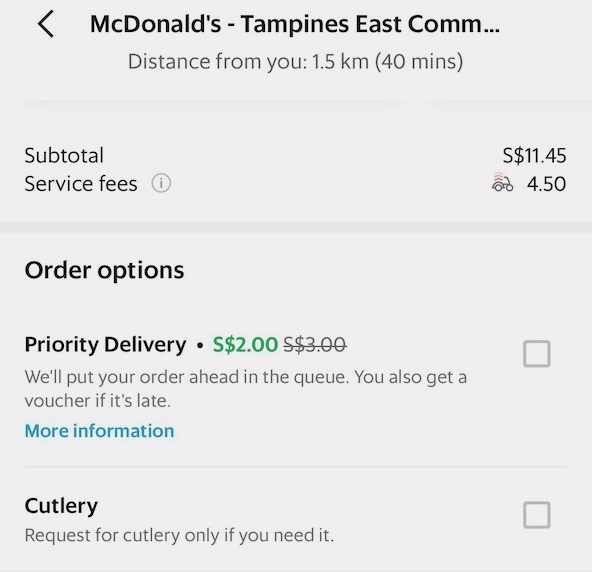The image is a screenshot of a segment from a food delivery app interface, specifically showcasing an order from McDonald's located at "Tampines East Com...". The screen indicates that the McDonald's branch is 1.5 kilometers away or approximately a 40-minute delivery time.

Displayed prominently is the order subtotal amounting to 11.45 Singaporean dollars (S$). The service fees are listed as 4.50 Singaporean dollars, accompanied by an information icon. Alongside this, there is a small icon resembling a scooter, possibly indicating the delivery method.

The order delivery options feature an unchecked box for "Priority Delivery" priced at a discounted rate of 2 Singaporean dollars from an original 3 Singaporean dollars. This option promises to prioritize the order in the delivery queue and offers a voucher if the delivery is late. More information about this option is available via a clickable link.

Another unchecked box is present for cutlery requests, encouraging users to request cutlery only if necessary.

The overall design is clean with sections divided by white boxes on a very light gray background, maintaining a minimalistic and user-friendly interface. No additional order details, buttons for confirming the order, or further interactive elements are visible in the image.